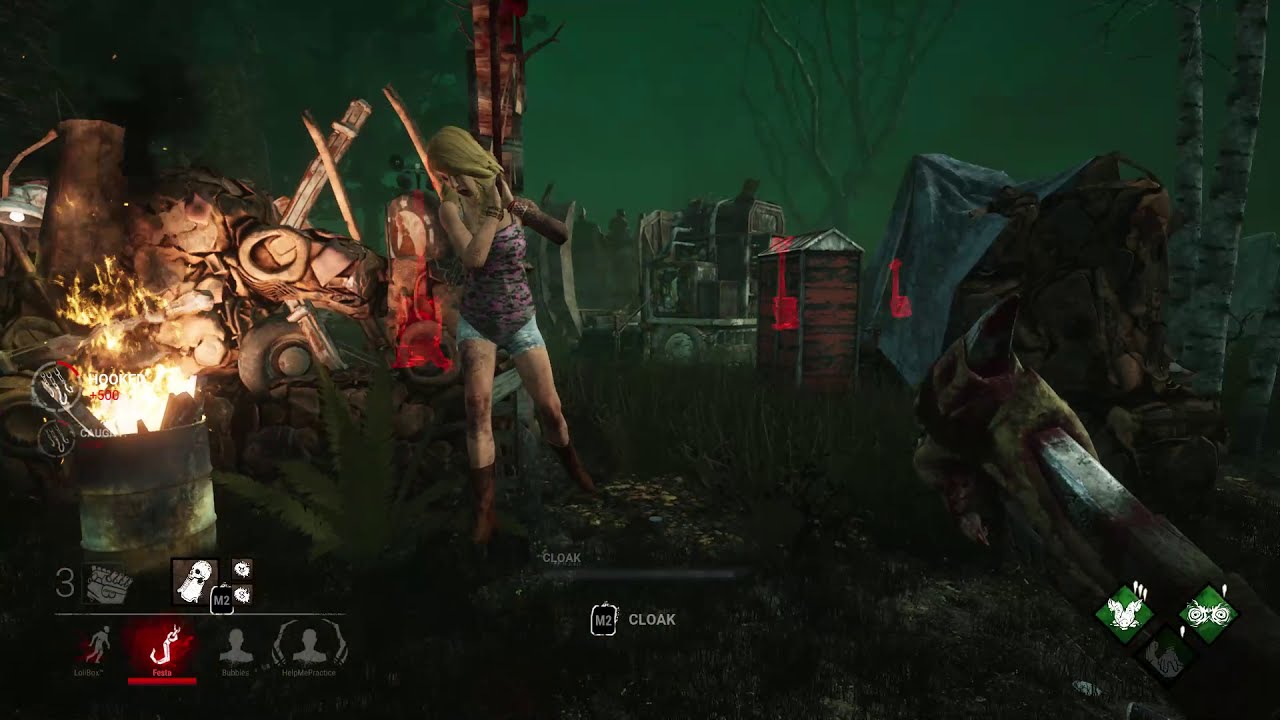The image is a vivid color screenshot from a video game, depicting a storage room setting that evokes the atmosphere of a junkyard or a post-apocalyptic scenario. The background is dominated by a green wall, and to the left of the scene stands a circular tall pocket overflowing with flyers. Behind this pocket lies a fenced area filled with various items, including circular objects resembling vehicle tires and long wooden poles. A woman, dressed in cutoff blue jeans and a multicolored top, sits on the fence. She wears high brown boots and has a green cloth covering her blonde hair. Her hands are raised, and though her face is only partially visible, she appears focused.

Also in the scene, on the left, a barrel with a burning fire emits a warm glow, contributing to the overall gritty environment. A metal bucket filled with wood on fire stands nearby, suggesting a makeshift heating or signaling method. The setting includes isolated clusters of junk, in varying shades of brown and gray, contributing to the desolate appearance. In the distance, a green hazy sky looms over a mix of trees, with one distinctly birch-like tree on the far right.

Scattered within the scene are objects and indicators suggesting this is a gameplay interface: translucent red bags, potential items to be collected, are strategically placed throughout the area. In the bottom corners of the image, there are in-game controls. The bottom left shows different characters alongside the word "cloak," while the bottom right displays two diamond-shaped icons representing weaponry and money. The meticulously designed setting, with its blend of survival elements and strategic gameplay objectives, immerses the player in a gripping and challenging virtual environment.